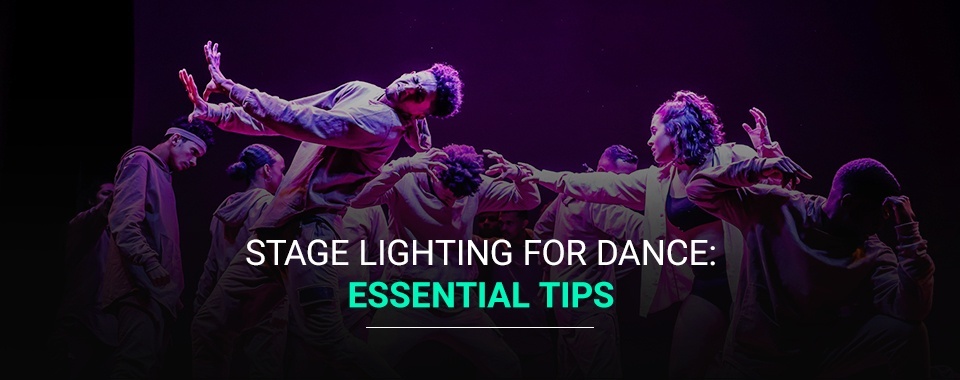This promotional banner, likely featured on an advertisement or a blog, is a long rectangular image filled with dynamic energy from a dance performance. The image’s text, positioned centrally at the bottom, reads "STAGE LIGHTING FOR DANCE: ESSENTIAL TIPS," with "ESSENTIAL TIPS" highlighted in a notable blue color, separated by a white line.

Set against a dark backdrop seamlessly blending from black edges into a deep purple center, the scene vividly captures the intensity of the dancers illuminated by a striking purple light that casts a glowing effect and emphasizes their movements. The group, consisting of around seven people, is engaged in various dance poses that convey a range of emotions and movements.

On the left, a short-haired man with a headband and a long-sleeve shirt appears to be in mid-movement next to a woman with a black ponytail, her back to the camera, wearing a hoodie. To their right, a front-facing man with a pained expression is stretching his arms out, dressed in a brown shirt and brown pants. Nearby, another dancer tilts his head forward, hands near his head as if grasping it, dressed in a long-sleeve shirt. Behind them, the top of a man’s head is visible, suggesting action in the background.

Continuing right, a woman in a sports bra and black panties, with shoulder-length hair, is reaching forward, wearing a long-sleeve shirt open in front. Further right in a shadowy area, another man is bent down with his left hand on his knee and his right arm extended back, adding to the dramatic composition of the scene framed with a subtle black vignette, enhancing the focal text.